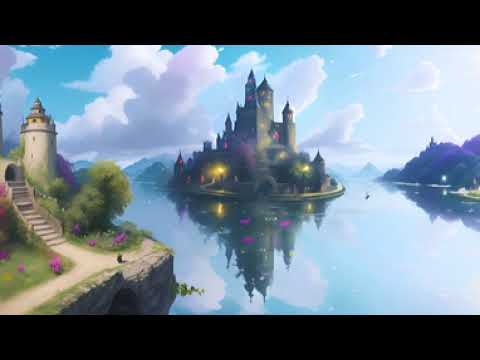The image depicts a fantastical, watercolor-esque or digitally generated scene showcasing a majestic castle situated on a circular island at the center of a vast lake. The castle, constructed in shades of gray with accents of purple and yellow lights, features numerous towers and spires, with the tallest ones crowning the center, forming a vaguely triangular silhouette. The lake beneath is pristine, mirroring the entire castle and creating a striking reflection of the structure and the fluffy white and bluish-purple clouds overhead, as well as the distant mountain range fading into the horizon.

In the foreground on the left side, a rocky land protrudes, leading up to a lighthouse-like tower atop a cliff, with a series of steps descending into a man-made cavern below. This area is dotted with pinkish-purple and green bushes, adding a touch of vibrant color against the greenery. On the right side of the scene, a line of large purple trees and patches of green grass are also mirrored in the lake, enhancing the symmetrical beauty of the scene, which is framed by a serene blue sky and whimsical clouds.